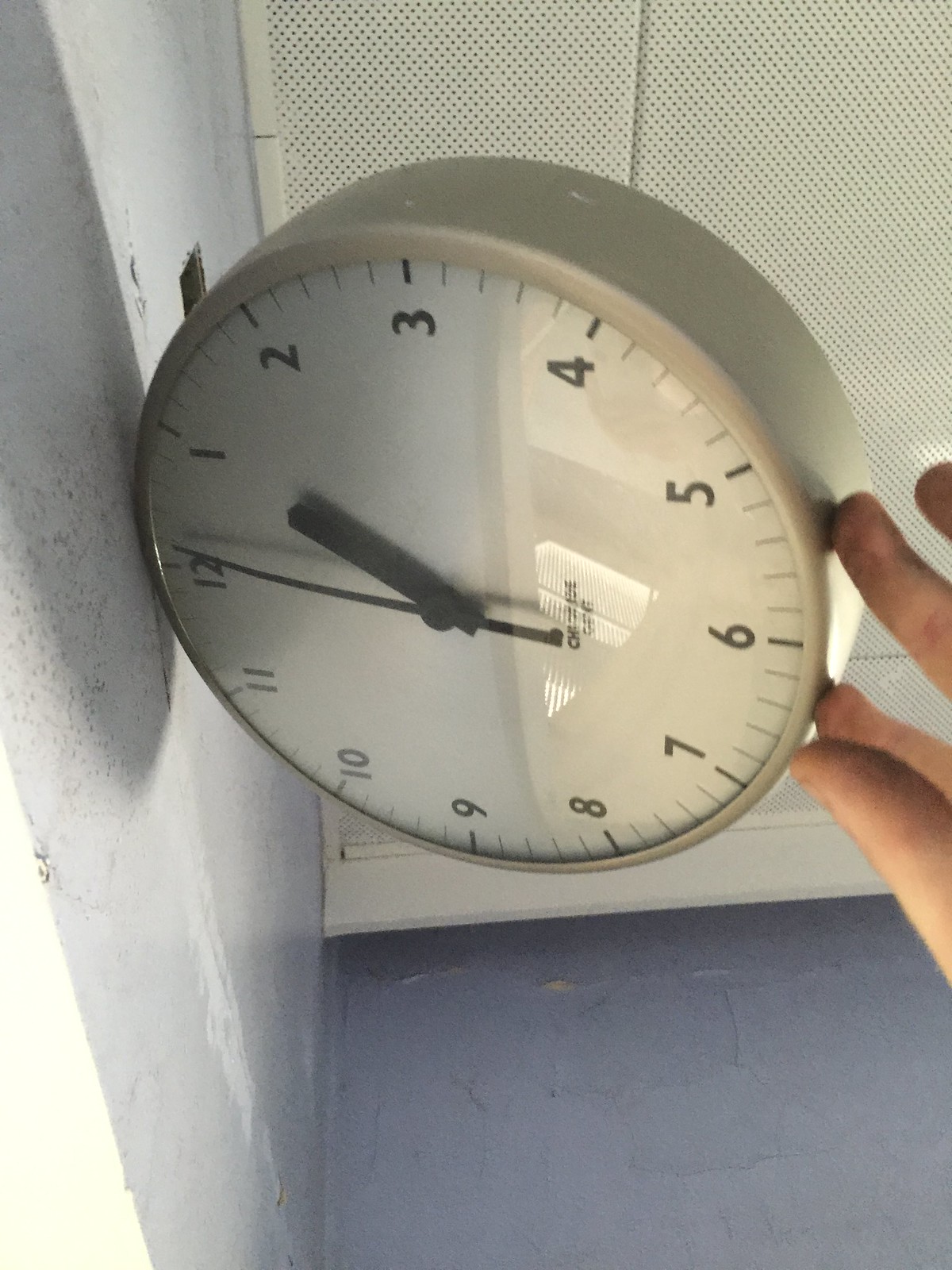The image features a scene layered with various textures and elements. On the right side, there is a stone wall with a white appearance and scattered black dots. In the background, a white wall metal merges with numerous small dots, and a depiction of a lion adds a focal point. The floor consists of stone, enhancing the overall rugged atmosphere. A notable feature is a reflective clock positioned towards the right. The clock face displays the numbers 1 through 12, with the minute hand pointing at 12 and the hour hand at 1. The casing of the clock appears to be made of a predominantly white metal. At the bottom of the clock, there is some text, though it's not clearly legible in the image.